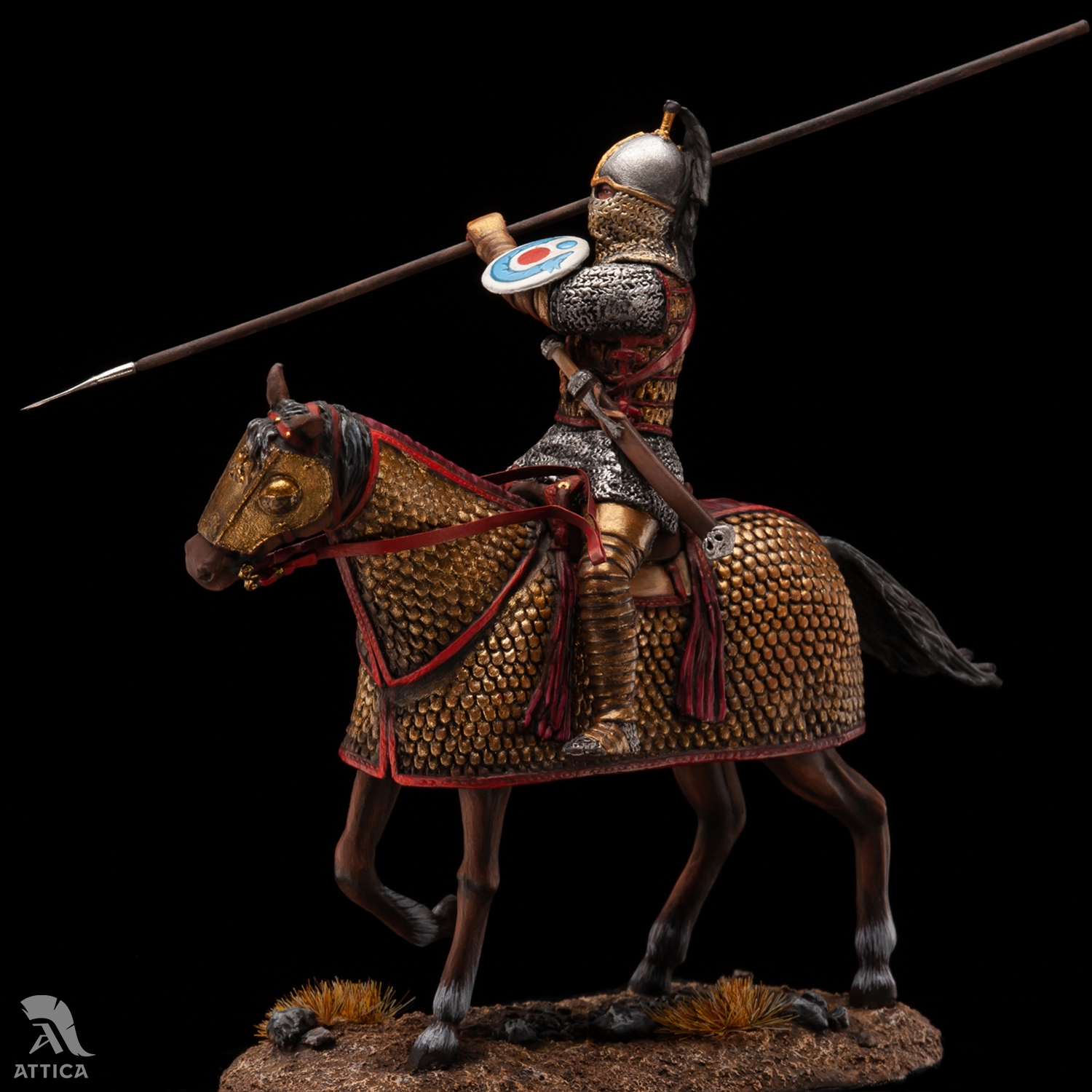The image depicts a detailed, up-close shot of a toy model set against a black background. Central to the scene is a knight mounted on a horse, both adorned in gleaming gold armor. The knight wears a helmet, accentuated with a small band, and dons mesh armor in silver and gold hues. He is equipped with a shield featuring a red center and blue edges, as well as a long spear with a wooden shaft and a silver tip. The horse's gold armor is detailed with red outlines and small stitches, enhancing its regal appearance.

Beneath the knight and horse, the terrain resembles a miniature desert landscape with small rocks, a few tufts of grass, and elements reminiscent of tumbleweeds. At the very bottom left corner of the image, the word "Attica" is displayed in white lettering. This intricate diorama captures a scene of chivalric grandeur, frozen in time.